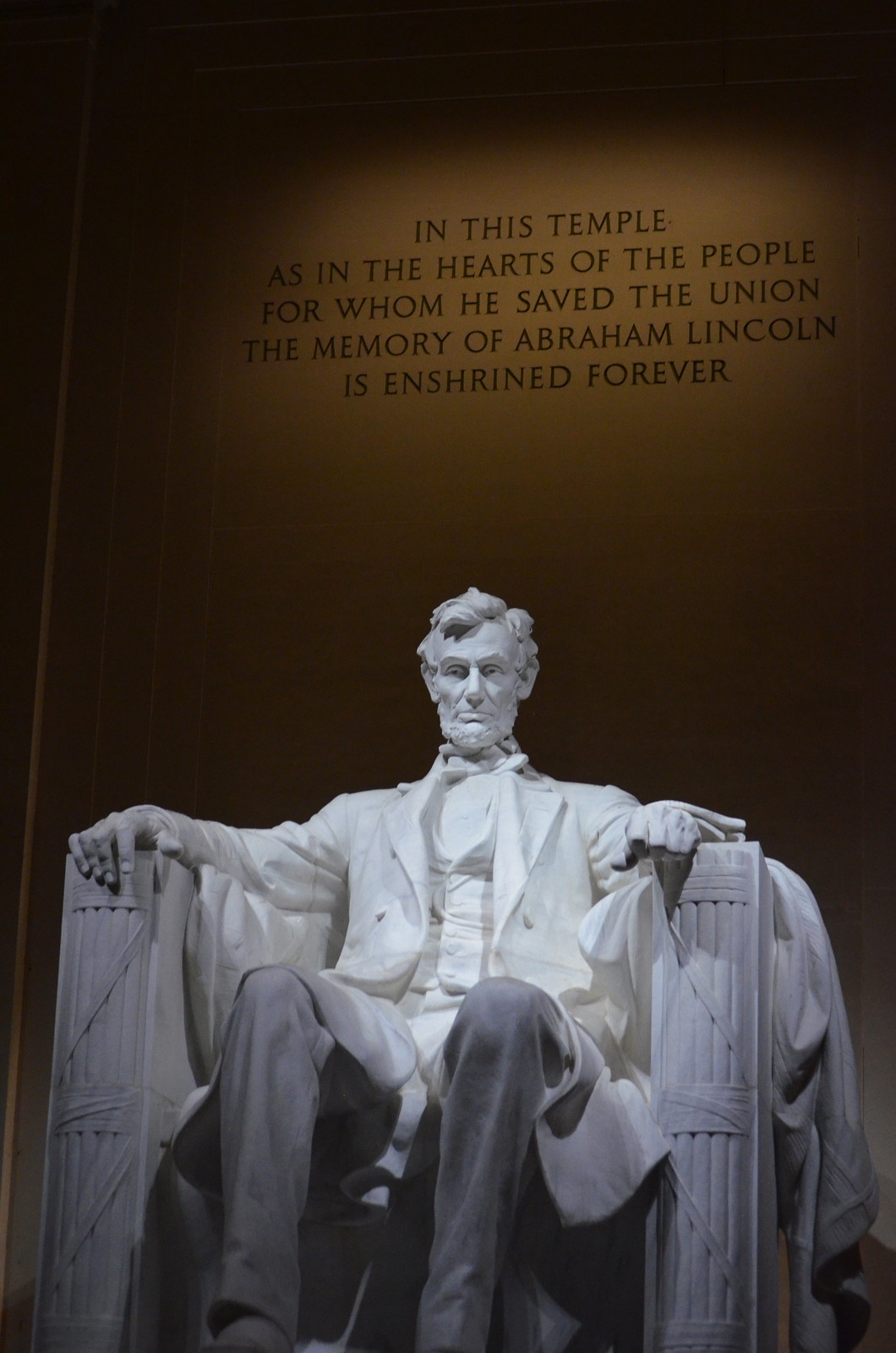This image depicts the famous stone statue of Abraham Lincoln, seated majestically on a colossal chair in Washington, D.C. The statue, carved from white stone, exudes meticulous detail, showcasing the textures of Lincoln’s coat, his neatly styled hair, and his hands resting on the armrests. His coat flows gracefully down, mirroring the drape of his pants. Behind Lincoln, a brownish backdrop is illuminated by a beam of light, highlighting the inscription in bold black lettering that reads, "In this temple, as in the hearts of the people for whom he saved the Union, the memory of Abraham Lincoln is enshrined forever." The overall composition captures the solemnity and reverence of this iconic memorial, with Lincoln's calm expression further emphasizing his enduring legacy.